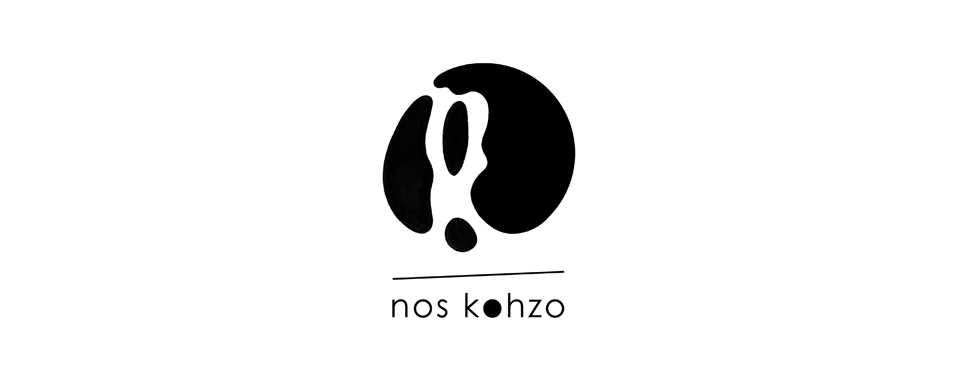The image appears to be a logo or graphic, characterized by its black and white color scheme. Against a white background, the centerpiece is a black abstract shape similar to an exclamation point, potentially reminiscent of a Rorschach inkblot. The central element consists of a long vertical black oval flanked by two crescent-like black blobs, with the left being slightly subtler in shade than the right. Just below the central figure is a small black circle. Underneath this arrangement is a thin horizontal black line that slants very slightly upward to the right. Below this line, in black lowercase letters, reads the text "noskohzo," where the first 'o' is distinctively filled in black. The overall design evokes a sense of modern minimalism, and the details suggest it could be a brand or product logo.